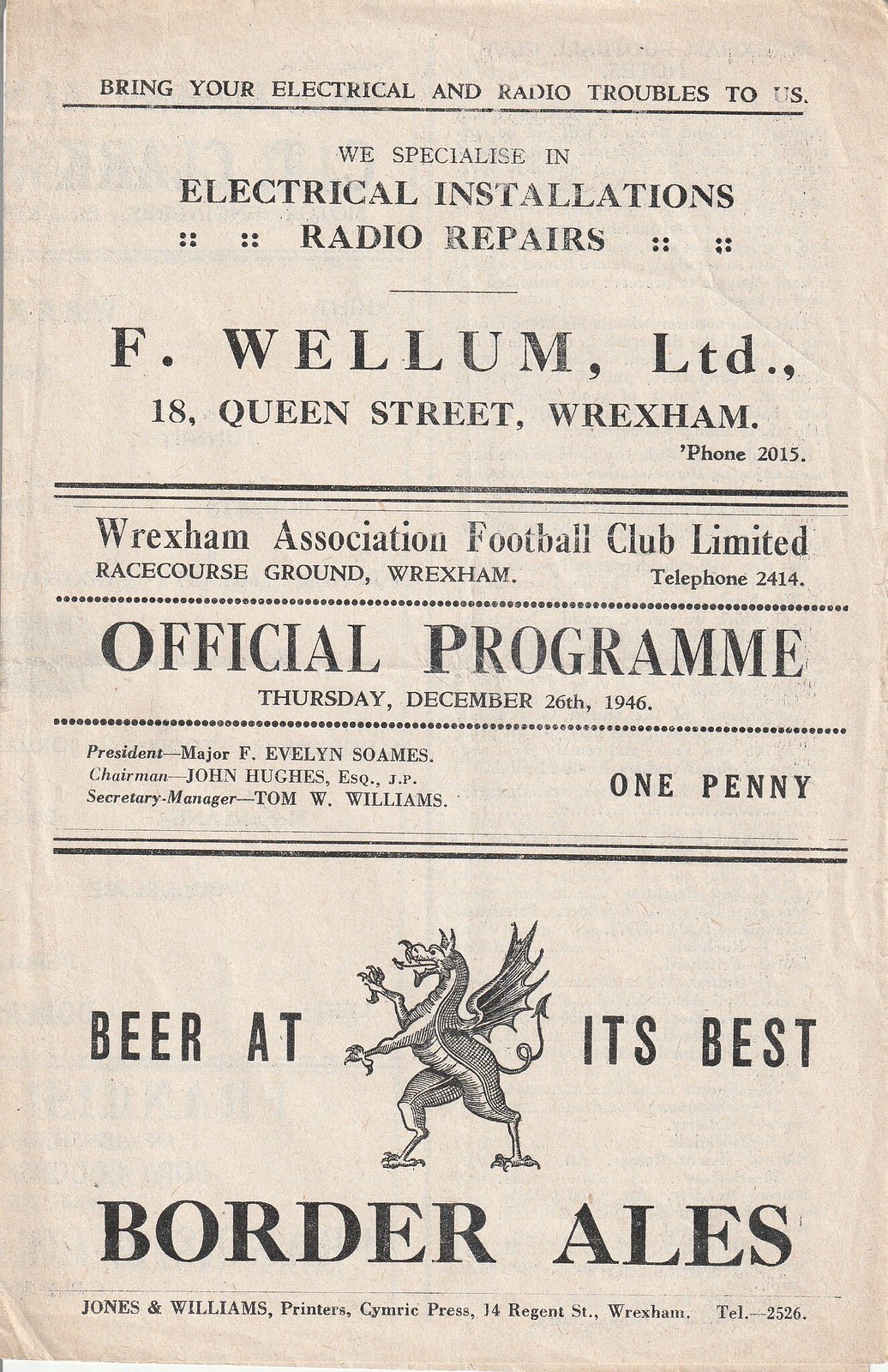The image is a black and white, vintage newspaper-style program, printed on cream-colored parchment paper. The promotional flyer occupies the top third of this program, crafted from gray-colored picture paper. At the top, in bold black English font, the flyer reads: "Bring Your Electrical and Radio Troubles to Us." Following this statement is a solid black dividing line. Beneath it, the text continues with: "We specialize in Electrical Installations and Radio Repairs." Another thin black line separates this portion from a line that reads: "F. Wellum Limited, 18 Queen Street, Wrexham, phone 2015."

The program itself dates back to Thursday, December 26, 1946, and lists its price as one penny. The bottom third of the page contains an advertisement for Border Ales, prominently featuring a large dragon logo with the phrase "Beer at its best" on either side of the dragon, emphasizing the vintage printing style of the overall publication.